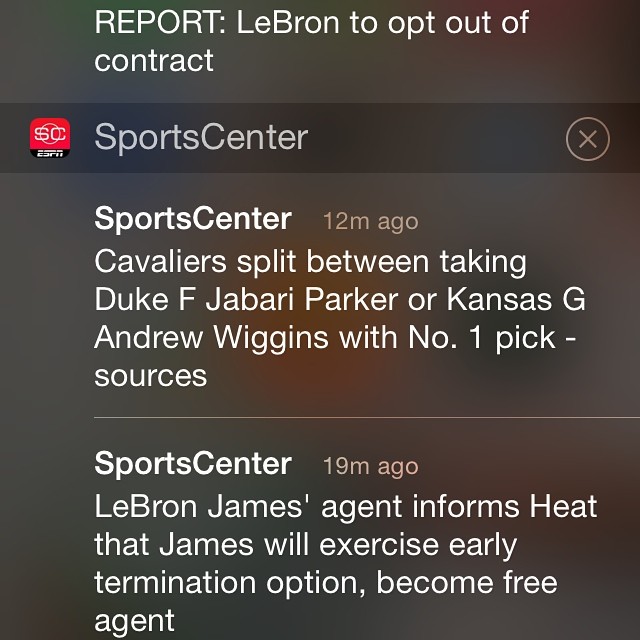The image depicts a screenshot of a phone notification from the SportsCenter app. At the top of the screen, the main headline reads "REPORT: LeBron to opt out of contract," set against a background with the SportsCenter logo and an 'X' icon indicating an option to close the notification. Beneath this, two recent updates are visible: 

1. A notification from 12 minutes ago states, "Cavaliers split between taking Duke forward Jabari Parker or Kansas guard Andrew Wiggins with number one pick - sources."
2. Another notification from 19 minutes ago reads, "LeBron James' agent informs Heat that James will exercise early termination option and become a free agent."

The notifications suggest a significant period in NBA history, possibly around 2013, when there was much speculation about LeBron James' future with the Miami Heat and potential draft picks for the Cleveland Cavaliers.